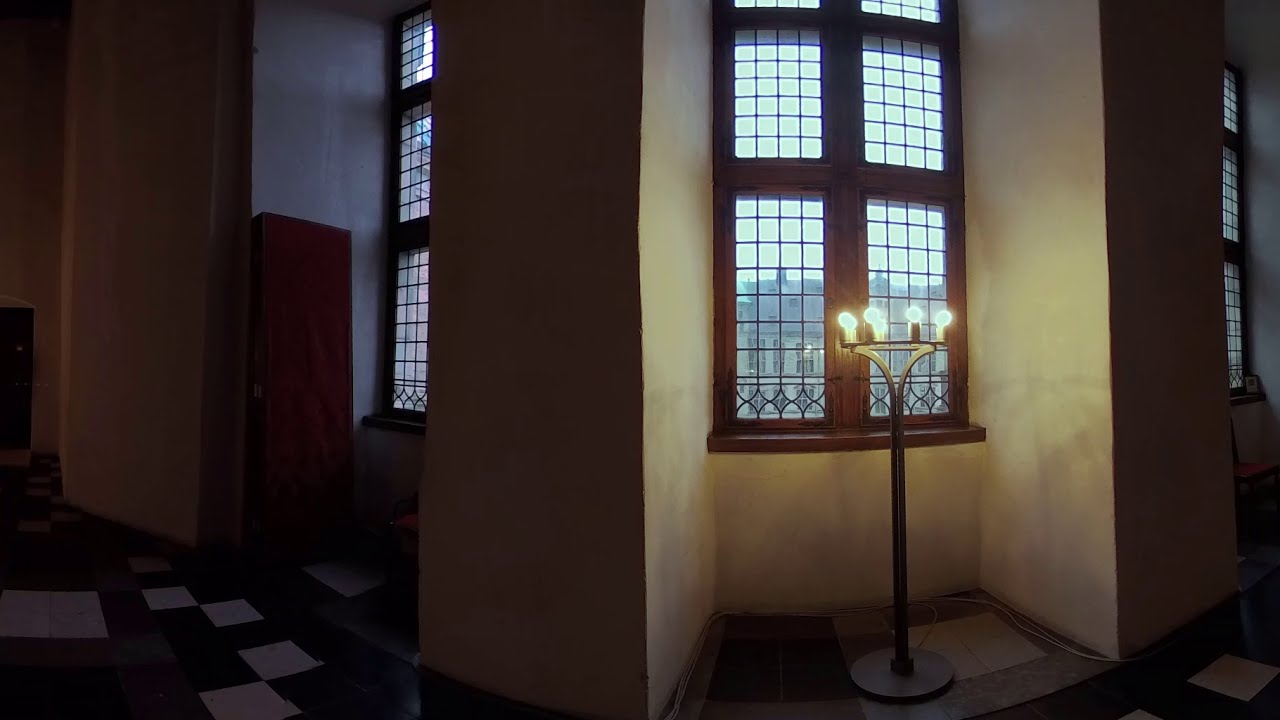The image depicts a slightly distorted panorama shot of a dimly-lit hallway, presumably in a church or cathedral, with a higher elevation offering a view of other buildings through latticed windows. The windows, although not stained glass, are segmented into small square panels, creating a grid pattern. To the right of the frame, there is a small alcove housing a stand with four lights arranged in a candle-like setting, which serves as the primary light source, casting a warm glow. The stand is approximately four feet tall and situated directly in front of a window. Pillars, brown in color, flank the stand on either side, extending from floor to ceiling and separating the windows. The hallway's floor features a black and white checkered pattern, adding to the ornate and traditional ambiance of the setting. The outdoor scene appears cloudy, as minimal light penetrates through the windows, enhancing the dimness of the indoor space.